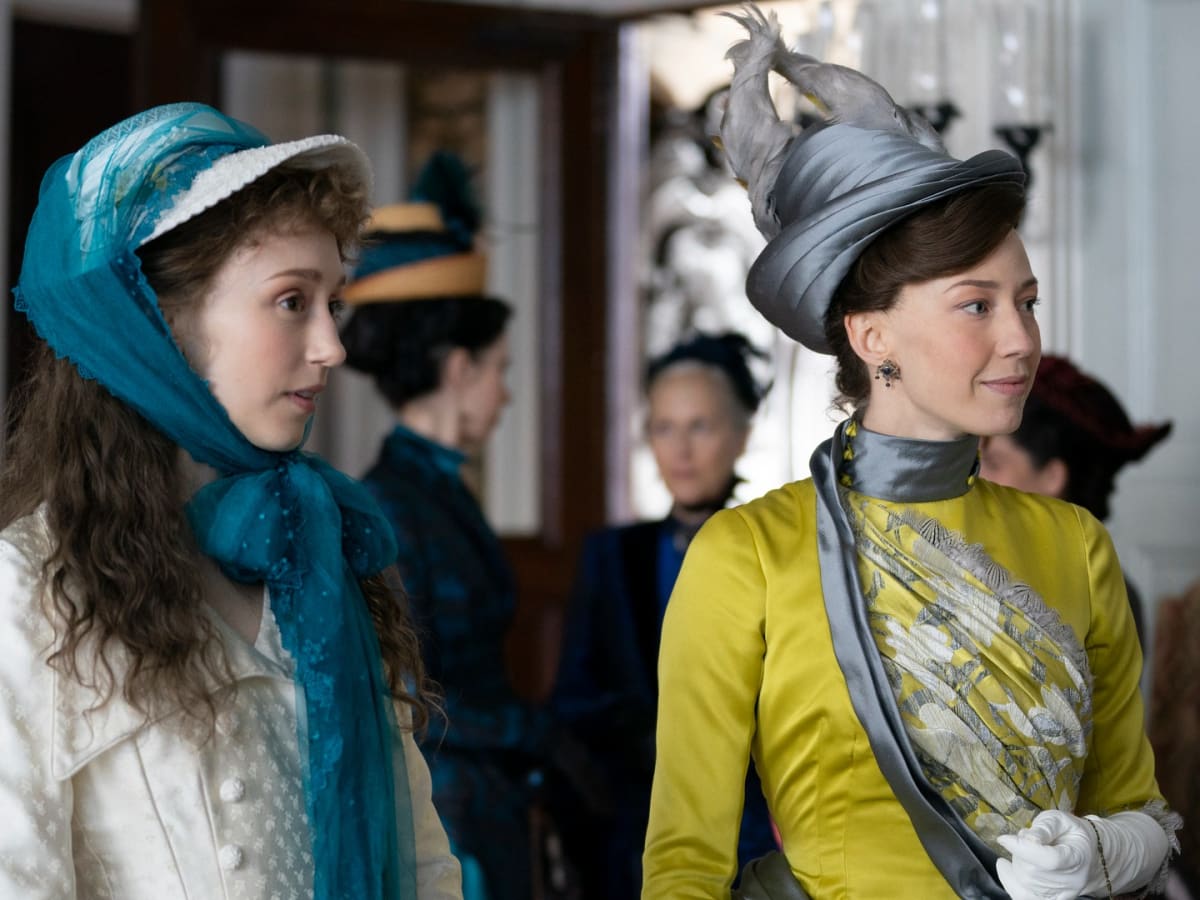In this detailed scene, likely from a period piece set in late 18th or early 19th century England, we observe a group of elegantly dressed women, seemingly attending a high-society event, possibly the Derby. The photograph is taken indoors during the daytime. 

In the foreground, two young women in their twenties capture our attention. The woman on the left wears a white dress with buttons and a white petticoat. Her ensemble includes a voluminous blue scarf tied under her chin, with long brown curly hair partially hidden under a white bonnet adorned with a veil and a ribbon hanging down her front. 

Her companion, standing to her right, is dressed in a light green, fitted dress, elaborately detailed with a white or silver applique and lace at the edges, possibly featuring a motif that resembles fish. She is accessorized with an intricate gray hat topped with feathers or bird wings, her brown hair styled in an updo tucked beneath the hat. She also wears a thin gray satin scarf, white gloves, and an ornate earring.

In the background, three women, blurred and out of focus, add to the scene's depth. They are dressed in darker hues, predominantly blue. The center woman's tall, ornate hat may be a visual effect created by the draped background, while the others appear to wear black or perhaps straw hats with turned-up brims.

The overall setting of this photograph exudes an atmosphere rich with historical elegance and sophistication, capturing a moment steeped in the fashion and social customs of its time.